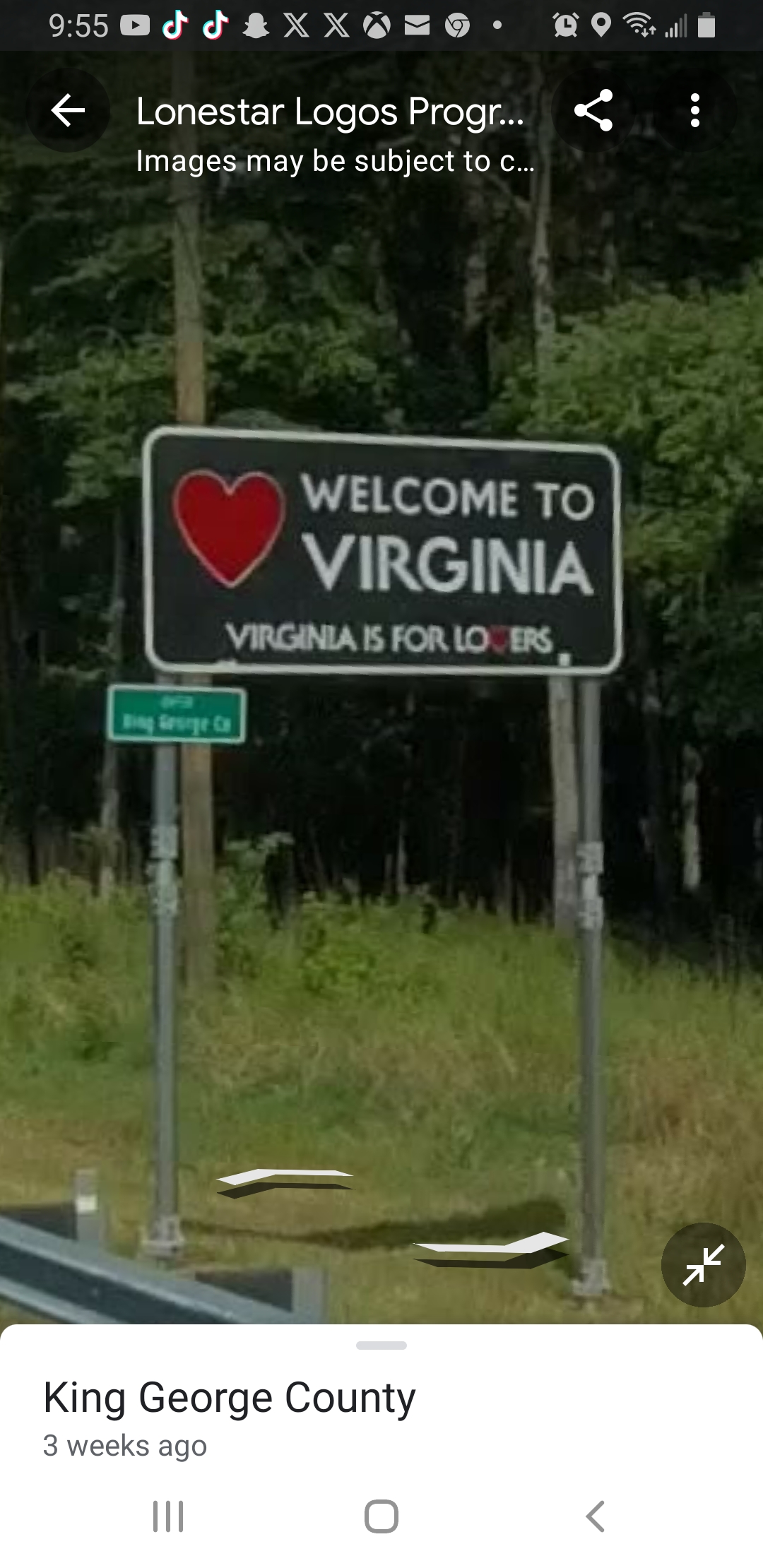The image features a close-up of a phone screen displaying two rectangular signs side by side. The smaller sign on the left is green with white text that is unfortunately illegible due to blurriness. The larger sign on the right has a white border and a black background. It prominently features a red heart on its left side and the text "Welcome to Virginia" on its right side.